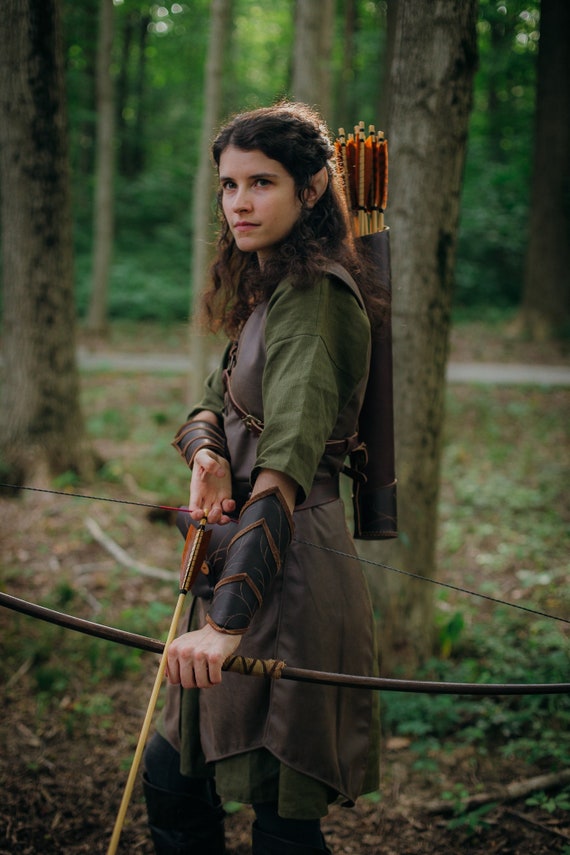In this detailed photograph, a woman is cosplaying as an elf and is shown standing in a forest, ready to shoot her bow. She has medium long hair pulled back, revealing pointy elf ear extensions. Her attire consists of a green top paired with a brown leather vest or tunic, a skirt, and high boots. She dons black leather bracers with pointed brown trim on her forearms. The woman grips a large bow in a semi-drawn position, with an arrow equipped, held between her index and middle fingers, and the top of the arrow resting on her left hand's knuckles. A quiver with seven or eight orange-feathered arrows is draped over her back in a leather holder. The forested backdrop is characterized by scattered tall trees and a mixture of green and brown ground cover, with a hint of a cement path visible in the background. The archer's serious expression and detailed attire, complete with the bow and arrows, create a vivid and immersive portrayal of an elf ready for action.